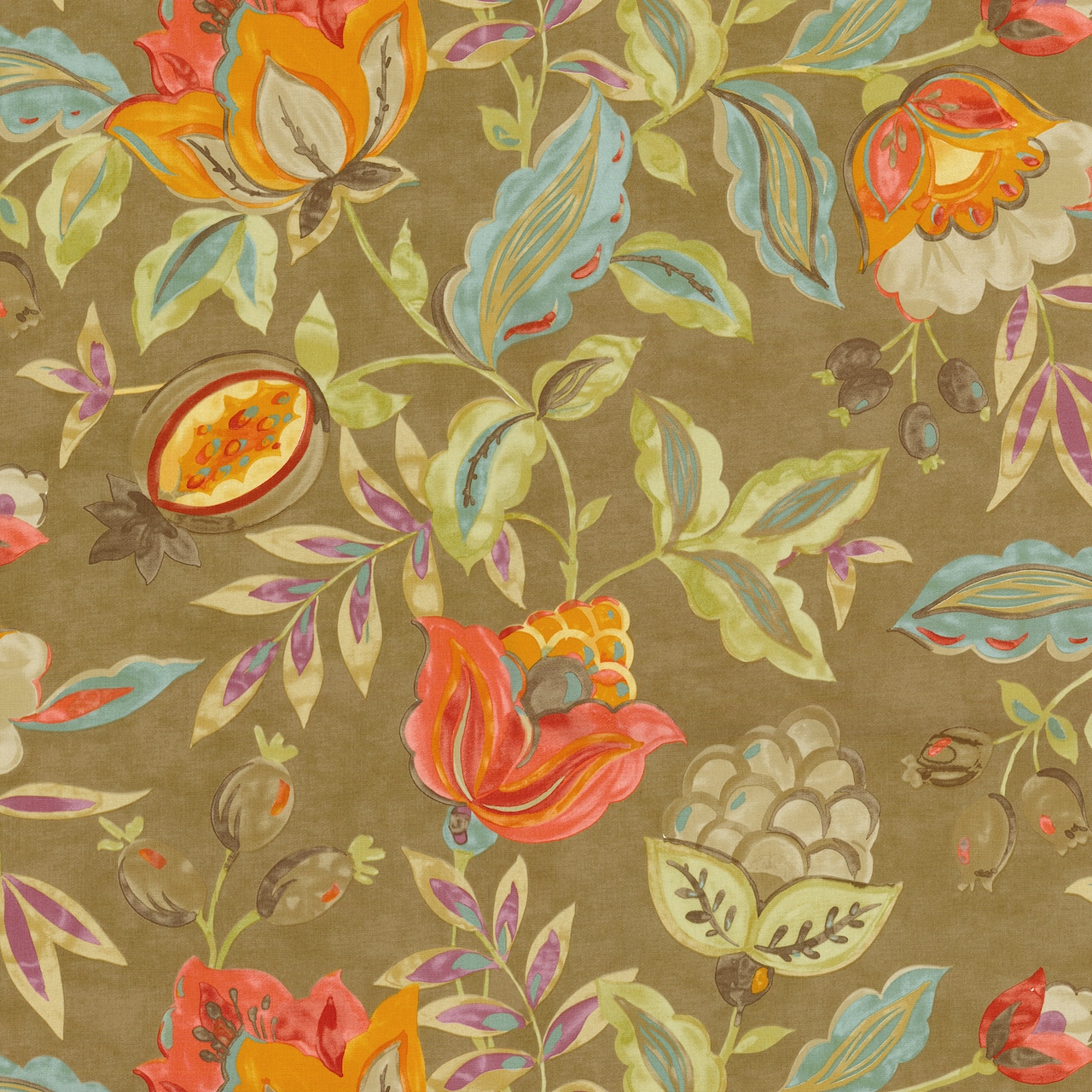This image is a detailed painting on a square canvas with a light brown, linen-like texture, reminiscent of a watercolor or spilled coffee stain, creating a varied tone background. The painting is an intricate composition of flowers and leaves spread across the canvas without any specific pattern. The flowers feature a warm, muted palette of red, burnt orange, light orange, yellow, and beige, blending seamlessly with the surrounding colors rather than standing out. Interconnected by delicate stems, the flowers are accompanied by triangular-shaped leaves in shades of beige, tan, purple, and blue. Scattered among the flora are small objects resembling fruit or olive-like buds. Notably, the top left corner showcases light blue petals with a light green center, while the top right corner features bright red petals with a darker brown leaf. In the bottom right corner, dark red petals paired with little brown leaves and a white fluffy flower emerge from a light green stem, and the bottom left-hand corner displays a faint arc of light blue. This intricate botanical print, possibly intended for wallpaper or fabric, combines various elements to create a cohesive yet vibrant brown and muted toned artwork.